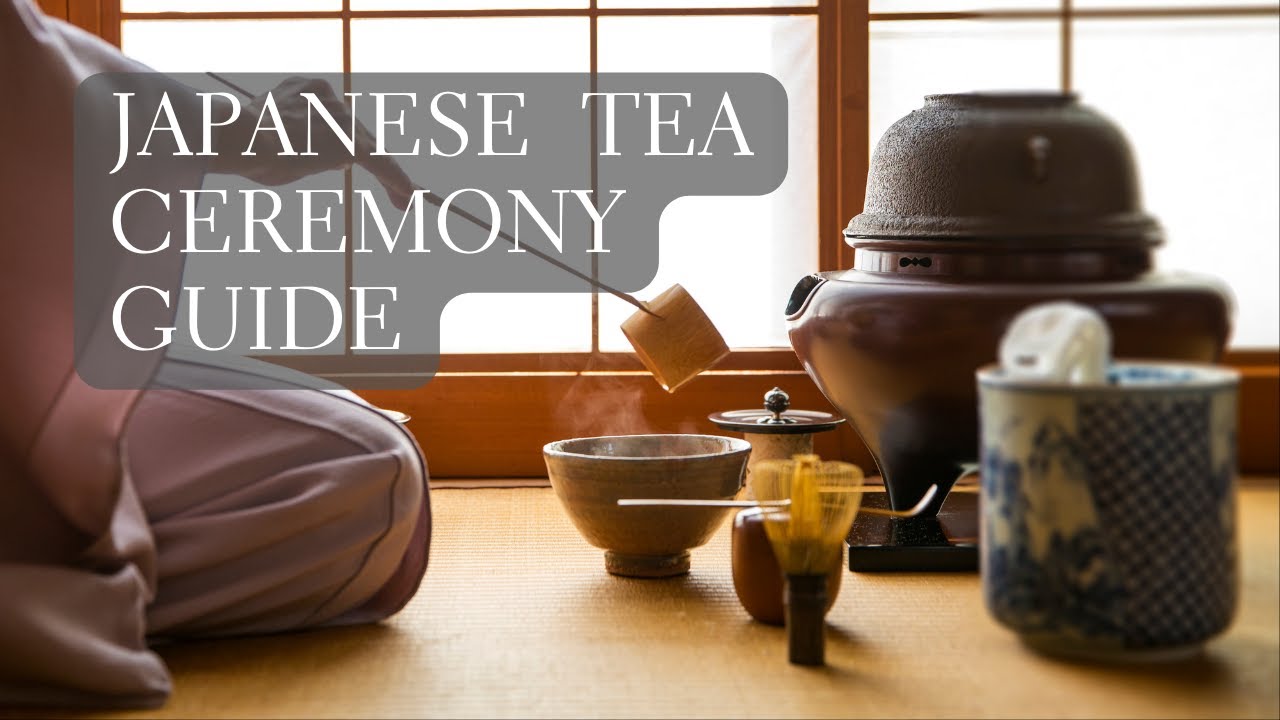The photograph showcases an intricately arranged Japanese tea ceremony scene within a traditional indoor setting. Dominating the image is the text "Japanese Tea Ceremony Guide" in a white sans-serif font, placed centrally towards the left. To the right of this text, a meticulously set-up tea ceremony arrangement is visible. The mahogany and dark brown tones of the tea set, combined with the beige and tan hues of the surroundings, create a warm and inviting atmosphere. A person, dressed in a light pink outfit, is kneeling on the left side, delicately dipping a teabag into a steaming brown pottery bowl, using a skewer. Nearby, a striking blue teacup adds a burst of color. The background is adorned with a traditional Japanese window screen, completing the authentic ambiance. The image features a palette of dark brown, black, blue, gray, beige, and transparent yellow tones, enhancing the overall visual appeal and traditional aesthetic of the Japanese tea ceremony.